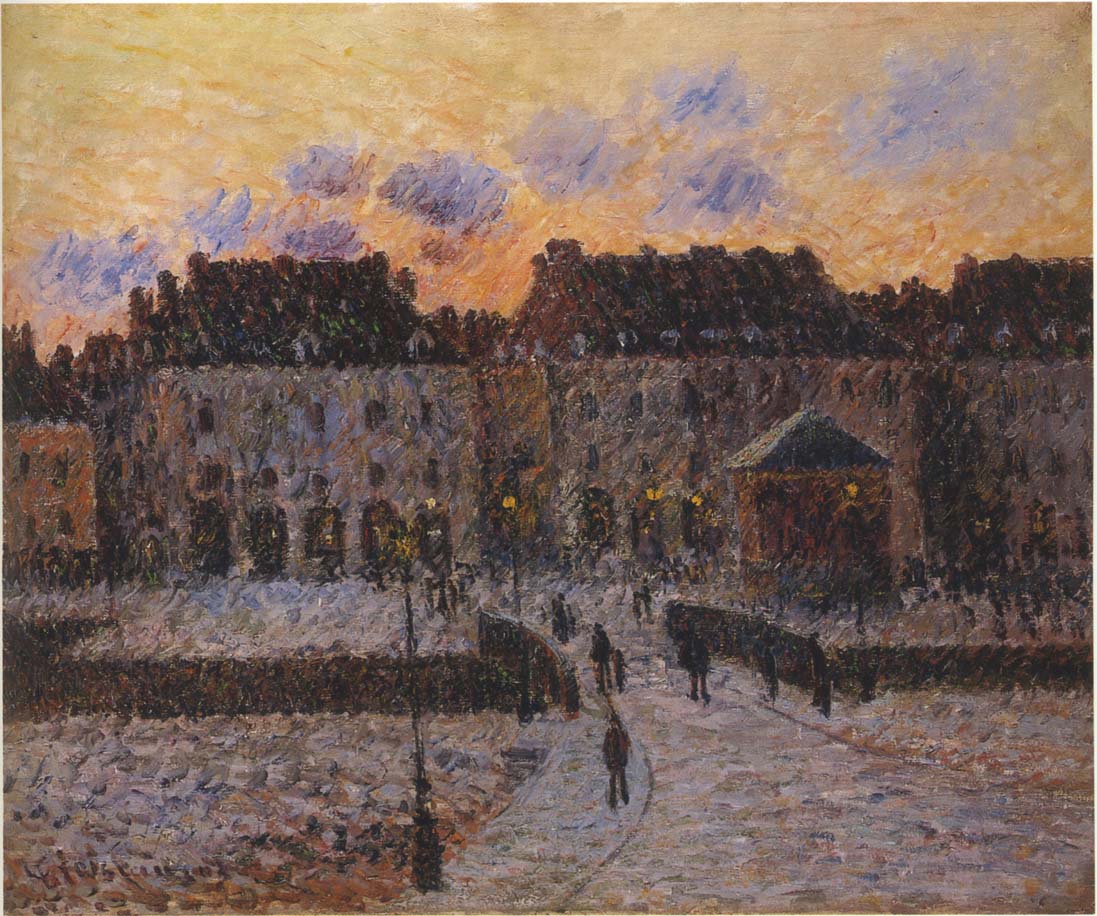This impressionistic painting portrays a bustling urban scene in a wintry setting. The sky, depicted in burnt orange and yellow hues with bluish-purplish clouds, suggests an early morning or late evening atmosphere. Beneath the vibrant sky, several three-story buildings with steep, dark-colored roofs and chimneys stand aligned, their whitish facades lining the street. The painting’s foreground features a snow-covered ground, accentuated by the abundance of white hues that dominate the canvas, separated from the background by a discernible fence. Streetlights illuminate the sidewalk where a man is seen walking, adding to the lively nature of the scene. A small bridge possibly crossing a canal is also part of the composition, contributing to the depiction of an active little town with numerous people engaged in their daily activities. The artist employs minimal brushstrokes, lending a blurred, almost shaky yet harmonious quality to the piece, emblematic of the French impressionist style.